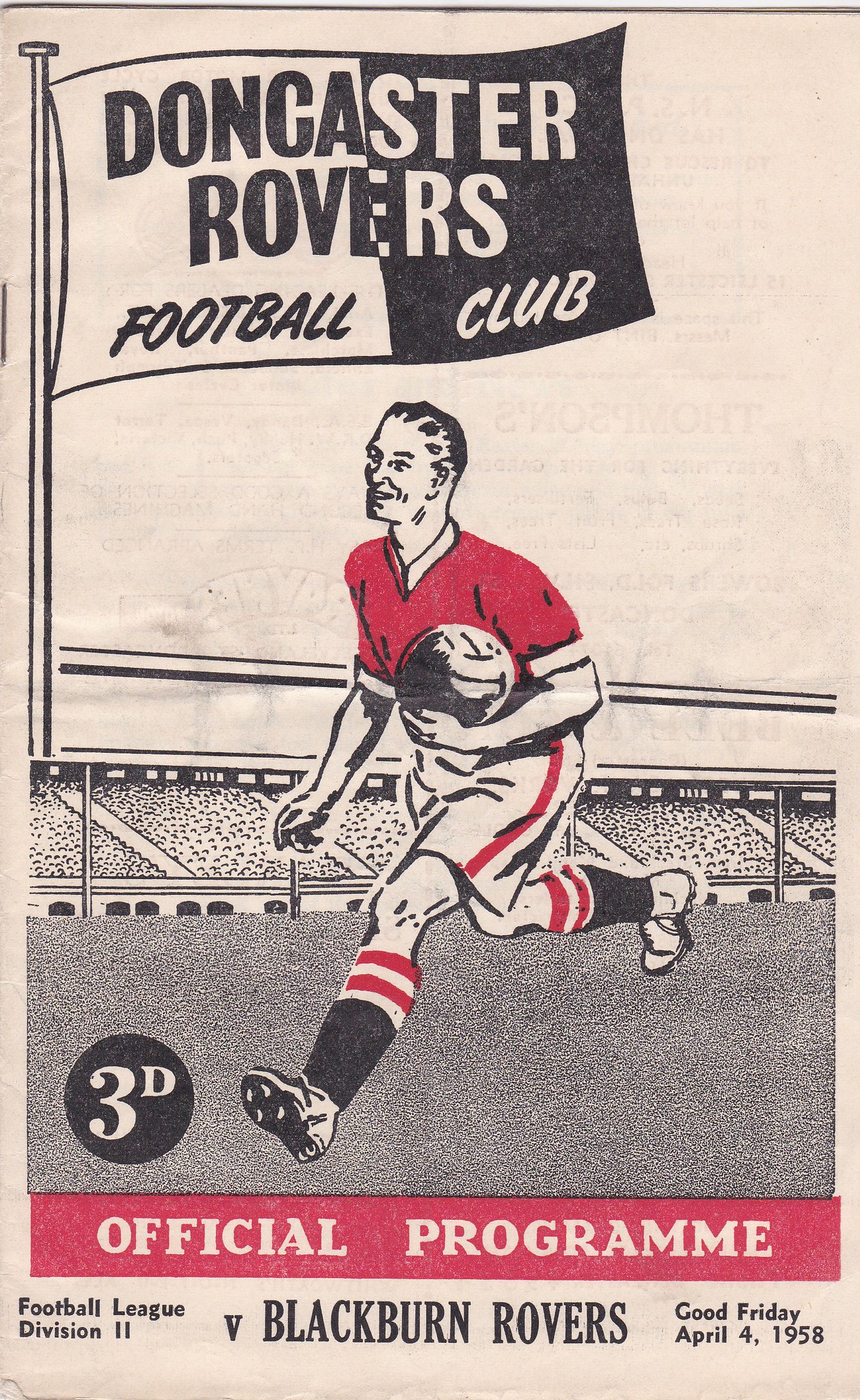This image showcases the cover of a soccer program from the Doncaster Rovers Football Club, set against a light pink background. At the top, a flag prominently displays "DONCASTER ROVERS" in bold capital letters followed by "FOOTBALL CLUB" in smaller, yet still all-capital letters. The flagpole appears on the top left and extends about halfway down the page. Beneath this, a soccer player dressed in a red and white uniform is depicted running with a soccer ball across a field. A representation of the stadium is in the background, illustrated with small curved marks to indicate spectators. At the bottom left, a circle encloses "3D," which likely represents the price of the program. Below this circle, a red section features the text "OFFICIAL PROGRAM." Near the bottom, larger letters announce a match between Doncaster Rovers and Blackburn Rovers, specifically labeled as a Football League Division 2 game. Finally, the date of the event, "Good Friday April 4th 1958," is prominently displayed at the bottom right.